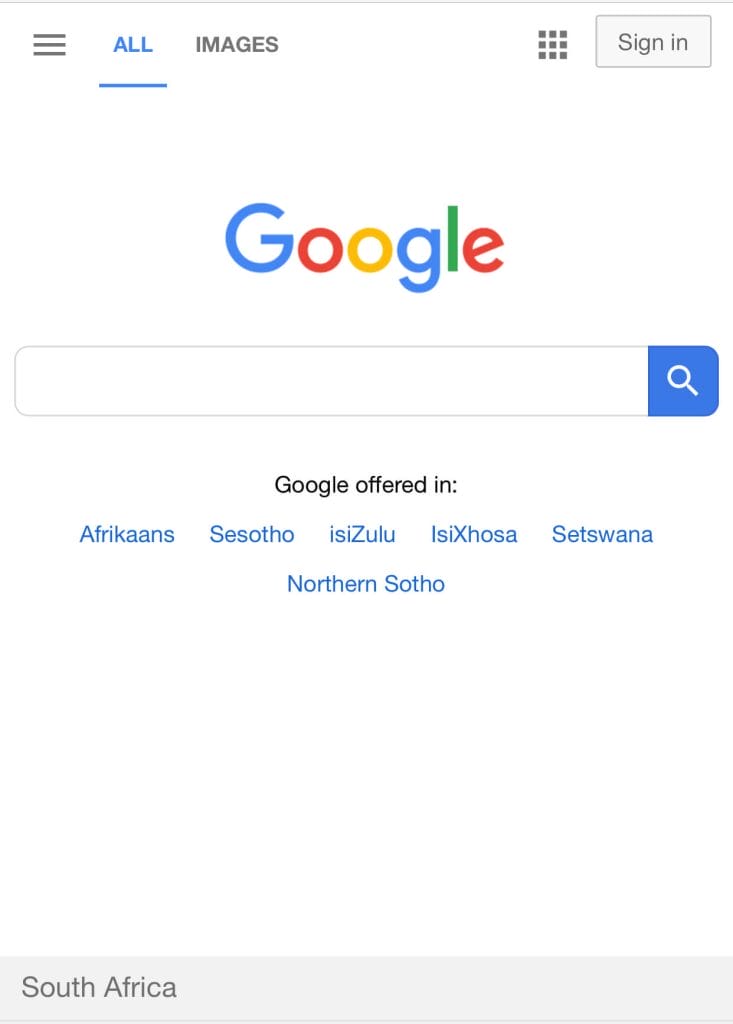A screenshot of the Google search engine's homepage. Dominating the center of the page is the iconic Google logo, immediately below which lies the search bar. At the far right end of the search bar is a blue section featuring a white magnifying glass, serving as the search button. 

In the top left corner, a 'hammer' icon is displayed, which, when clicked, reveals a list of additional options. Slightly to the right of this icon, the "All" tab is visibly highlighted in blue, indicating it is the selected option, with the "Images" tab situated next to it, shown in gray. 

At the top right corner, there is a 3x3 grid icon that leads to various Google applications when clicked. Adjacent to this grid icon is a 'Sign in' button, signaling that the user is currently not signed in.

Below the Google logo and the search bar, a line of text declares, "Google offered in," followed by a list of languages such as Afrikaans, Sesotho, isiZulu, isiXhosa, Setswana, and Northern Sotho, hinting at the user's location being South Africa, as further evidenced by the "South Africa" label at the bottom left of the screen.